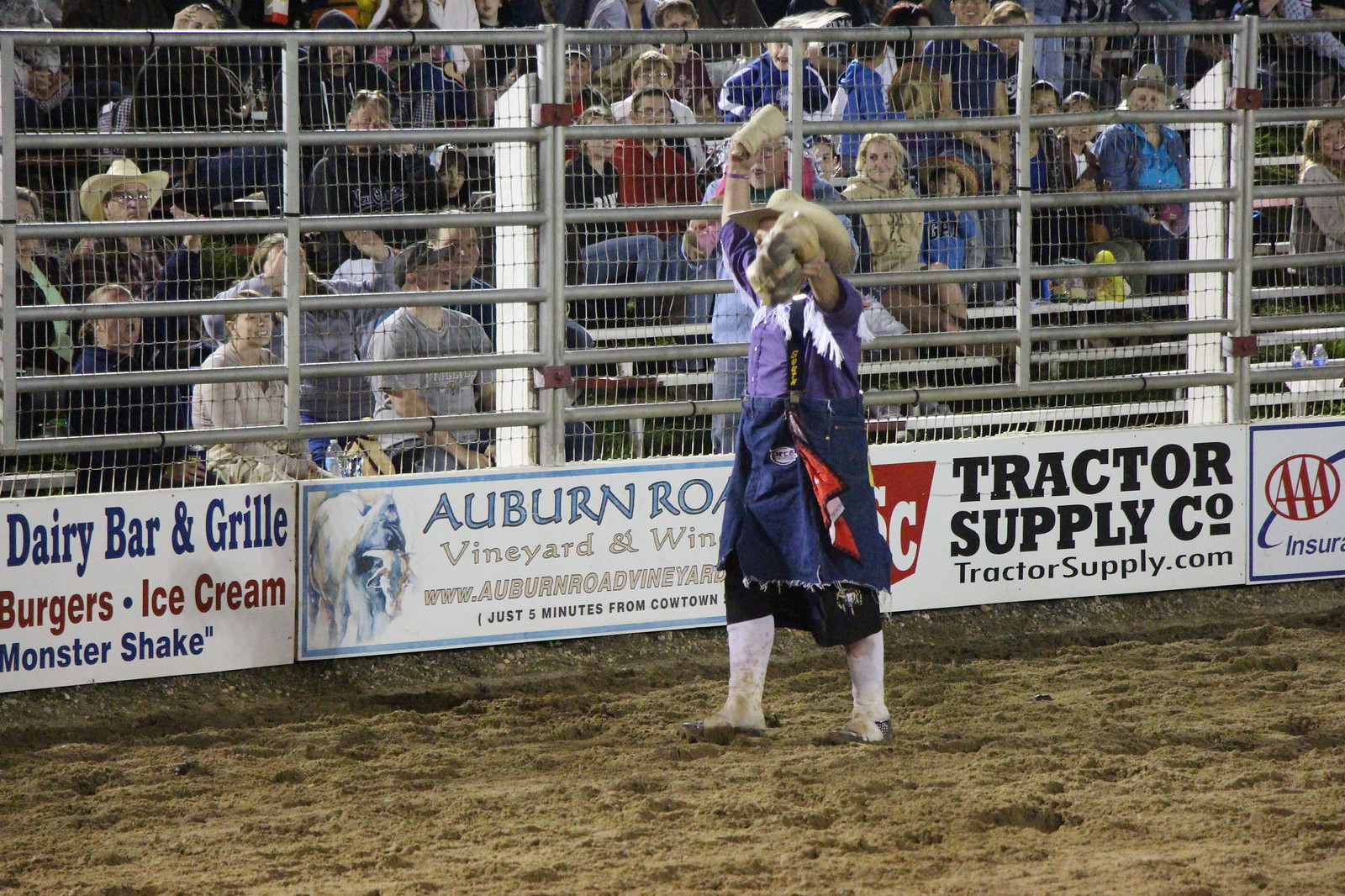In the center of a rodeo arena with a dirt floor, a rodeo clown dressed in an extravagant costume is engaging the audience. He is wearing a purple button-down shirt adorned with white tassels, oversized blue jean overalls cut off to resemble a layered skirt, tall socks, women's shoes, and a cowboy hat. The clown, possibly a bullfighter, is shaking a cowbell with his right hand and holding another object aloft with his left, possibly preparing to toss shirts or other items into the crowd. Surrounding the arena are various advertisements, including "Dairy Barn and Grill," "Burgers," "Ice Cream," "Monster Shake," "Auburn Road Vineyard," "Tractor Supply Company" at tractorsupply.com, and "AAA Insurance." Beyond the fence lined with these ads, a crowd—many wearing cowboy hats—watches the clown's antics, their faces lit up with smiles. The vibrant atmosphere captures the excitement and communal spirit of a rodeo event.